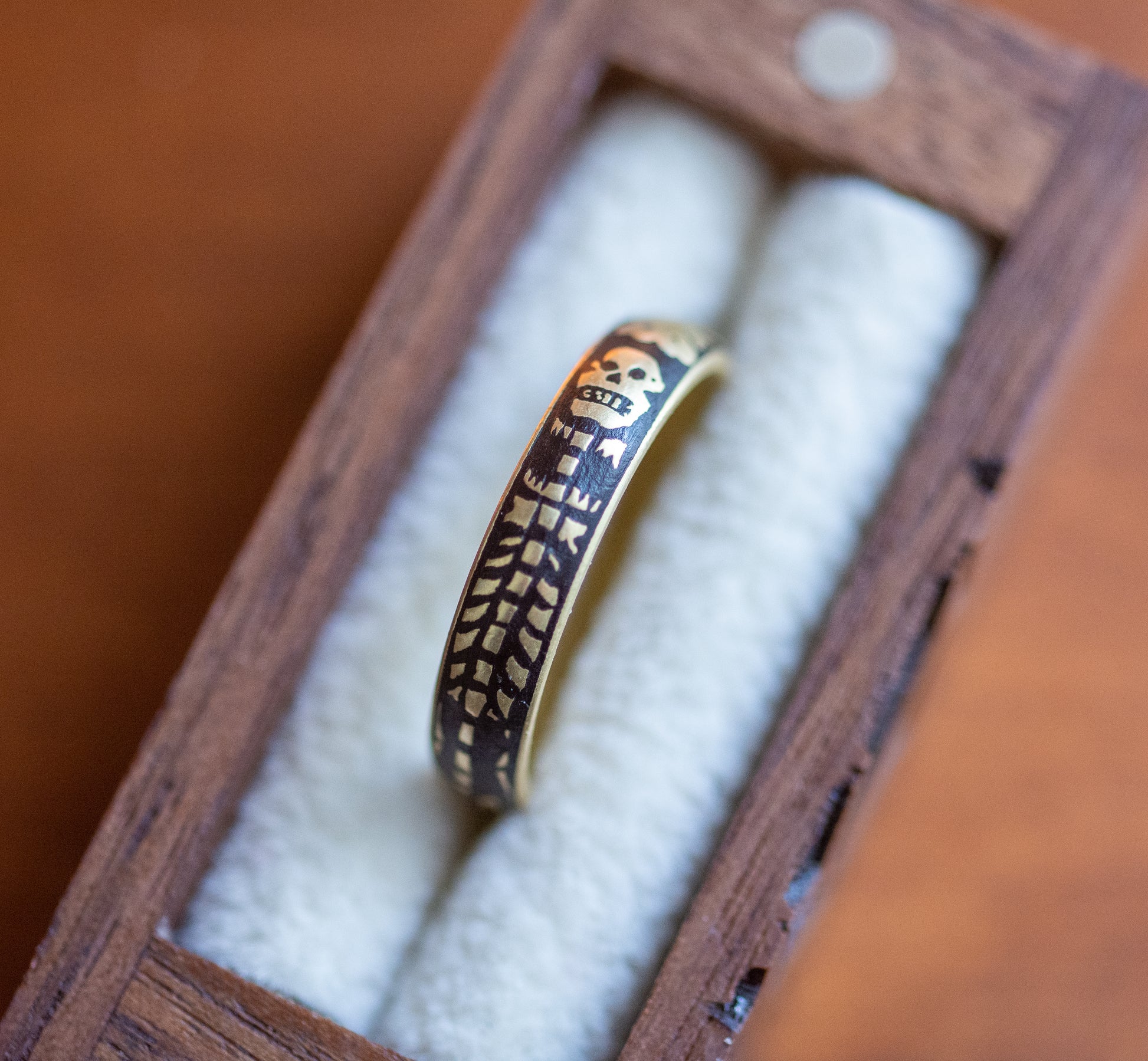The image is a slightly blurry photograph focusing on a distinctive gold ring with black detailing. The ring, adorned with an intricate gold skeleton design featuring a skull at the top and vertebrae and ribs along the band, utilizes negative space to highlight these details. The black segments emphasize the skeletal outline. The ring is securely positioned between two pieces of white cotton cloth within a light brown, textured wooden box. The background of the image appears to have a brownish, reddish clay earth tone, adding to the organic feel of the presentation. The setup suggests a sense of scale, with the small box enhancing the ring's intricate design and unique craftsmanship.